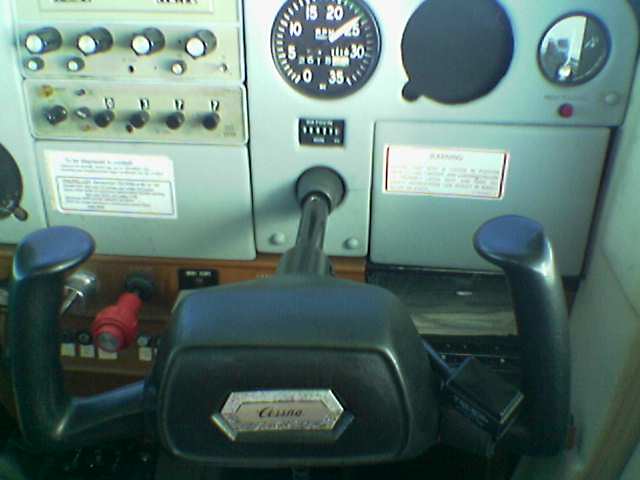This close-up image captures the detailed dashboard of a cockpit inside a small Cessna plane. Prominently featured is the steering wheel, extending from a gray metal panel, with two side handles that include thumb grips at the top. The wheel bears the Cessna logo on a silver background. Surrounding the wheel are various dials and displays, including a notable large black dial marked with numbers for precise readings. Additional circular dials, some with black casings and white tips, are scattered across the cockpit. A red knob stands out at the bottom left of the panel, which appears to be gold, contrasting with the gray metal of the rest of the cockpit. The scene is bathed in natural light, adding clarity to the details.